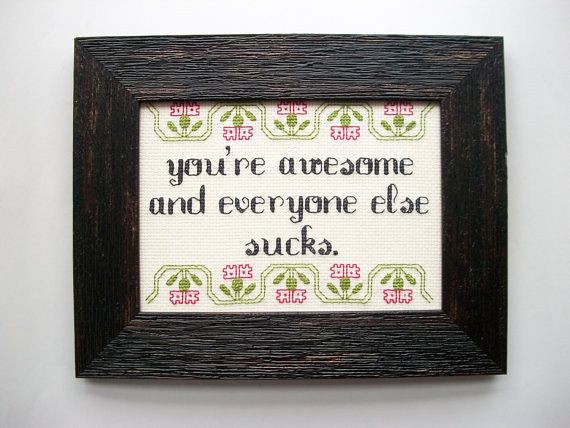The image showcases a meticulously crafted piece of framed embroidery art secured within a square, dark wood grain frame, likely around an inch and a half in width, and set against a gray background. The fabric inside the frame is white, adorned with intricately stitched designs. Predominantly, the embroidery reads, "You're awesome and everyone else sucks," in black script letters. Framing this central message is a border of alternating pink flower pots with three-leaved green flowers. These flower pot designs alternate directions, creating a dynamic up-and-down pattern both at the top and the bottom of the frame. The rustic, tactile frame enhances the handcrafted charm of the embroidered message and floral borders, creating a compelling and whimsical piece of art.